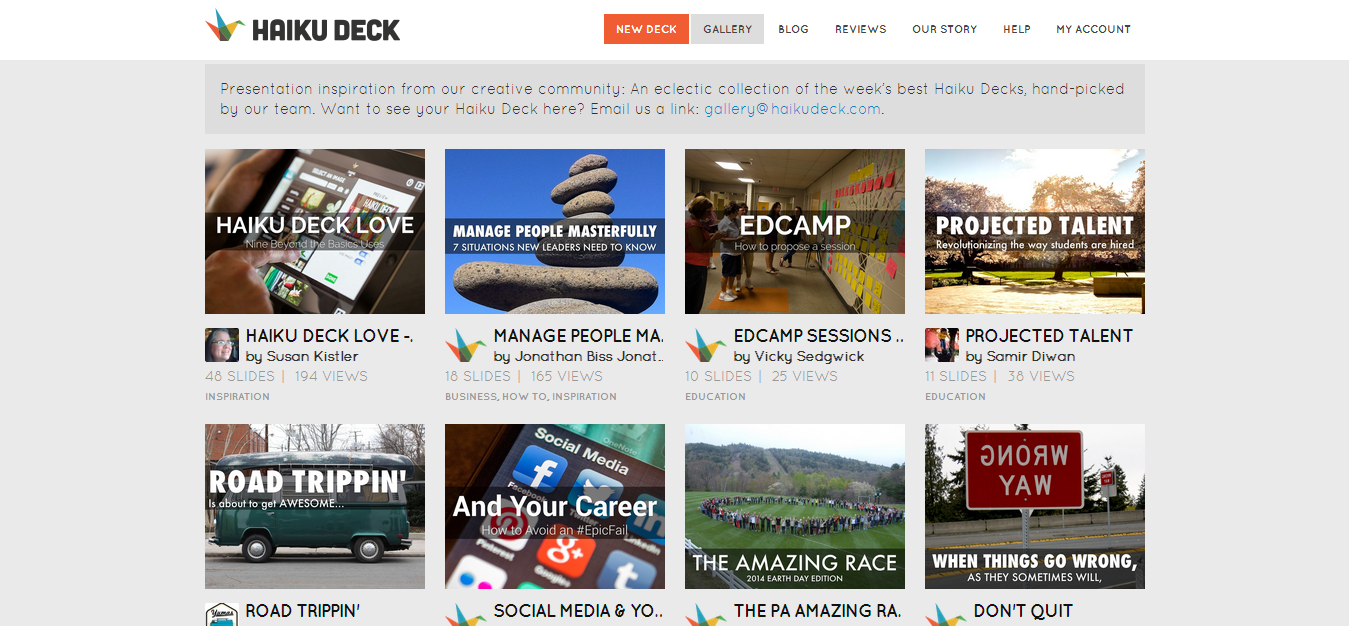This is the landing page of Haiku Deck's website. The top left corner prominently displays the Haiku Deck logo, which features a small origami bird. Along the top of the page, there are seven navigation options: "New Deck" (highlighted in red), "Gallery" (in gray), "Blog," "Reviews," "Our Story," "Help," and "My Account."

The main section of the page has a light gray background and showcases eight thumbnail images arranged in a grid of four on top and four on the bottom. Each thumbnail includes a title, an image, and a brief description below.

- The first thumbnail at the top left is titled "Haiku Deck Love," though the image and description are not specified.
- The second thumbnail, titled "Manage People Masterfully," features an image of stones against a blue sky.
- The third thumbnail, titled "Ed Camp," depicts people looking at a wall covered with sticky notes.
- The fourth thumbnail, titled "Projected Talent," shows trees with sunlight filtering through them.

On the bottom row:
- The first thumbnail, titled "Road Trippin'," features a picture of a bus.
- The second thumbnail, titled "And Your Career," displays a close-up of an iPhone.
- The third thumbnail, titled "The Amazing Race," shows a close-up image of many people standing in a circle.
- The final thumbnail, titled "When Things Go Wrong," features an image of a "Wrong Way" sign facing backwards.

Each thumbnail leads to a corresponding video or detailed description upon being clicked.